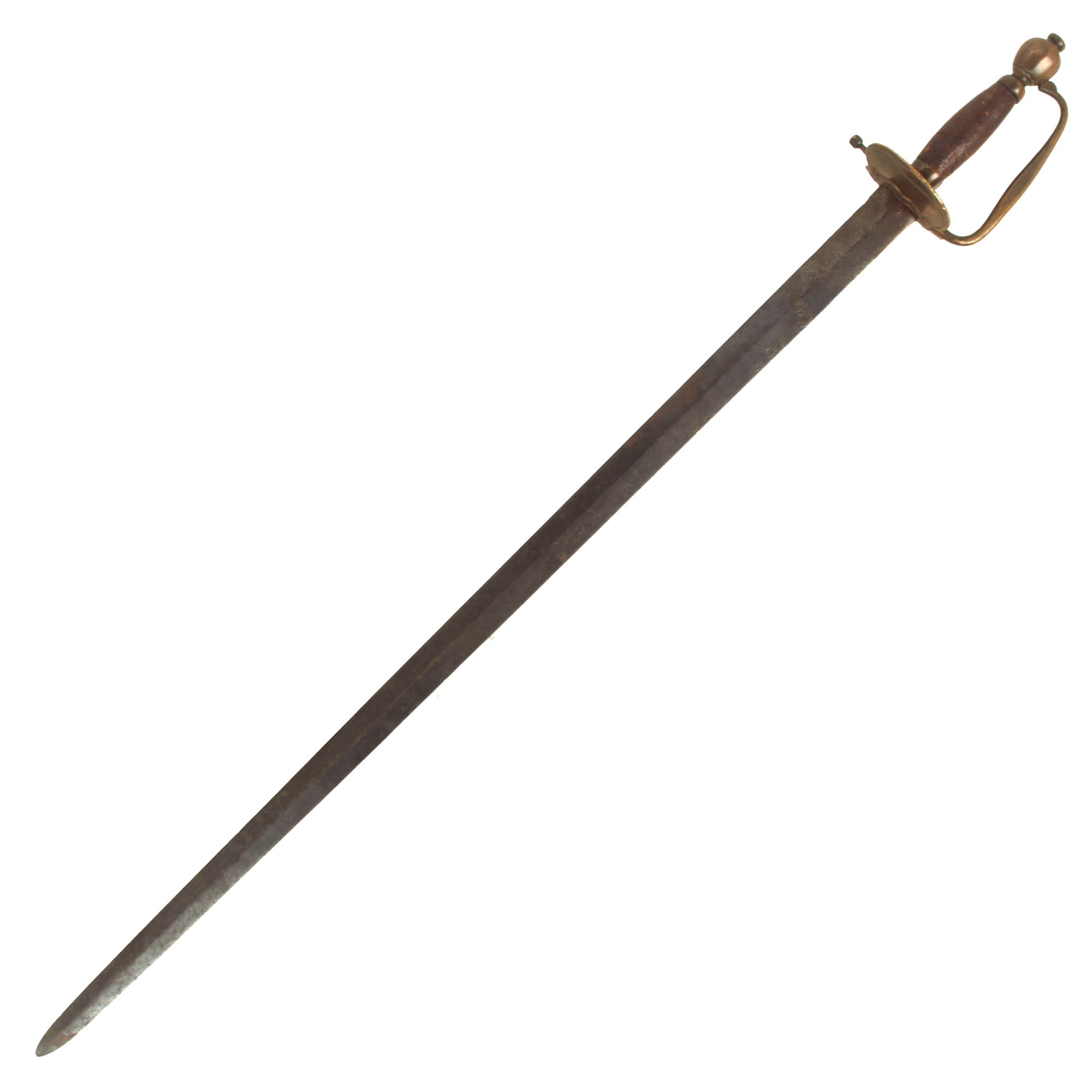The photograph captures a weathered, antiquated sword diagonally spanning the entire image, with its pointed tip aimed towards the bottom left corner and the pommel directed towards the top right. The blade, crafted from metal, exhibits a browned, aged appearance and is visibly dull and battered. The hilt, featuring a round circular crossguard and a C-shaped handguard, connects seamlessly to both the pommel guard and the crossguard. The blade transitions from a darker gray near the handle to a slightly lighter hue towards the tip. The handle, darker than the blade, is tinged in a brassy gold tone, while the knobs near the pommel bear a striking gold color. The sword is set against a stark, solid white background, emphasizing its presence as if it were floating in a void, and suggesting that the photograph might be intended for showcasing or selling the piece. The overall image is square-shaped with equal-length sides, contributing to its balanced composition.